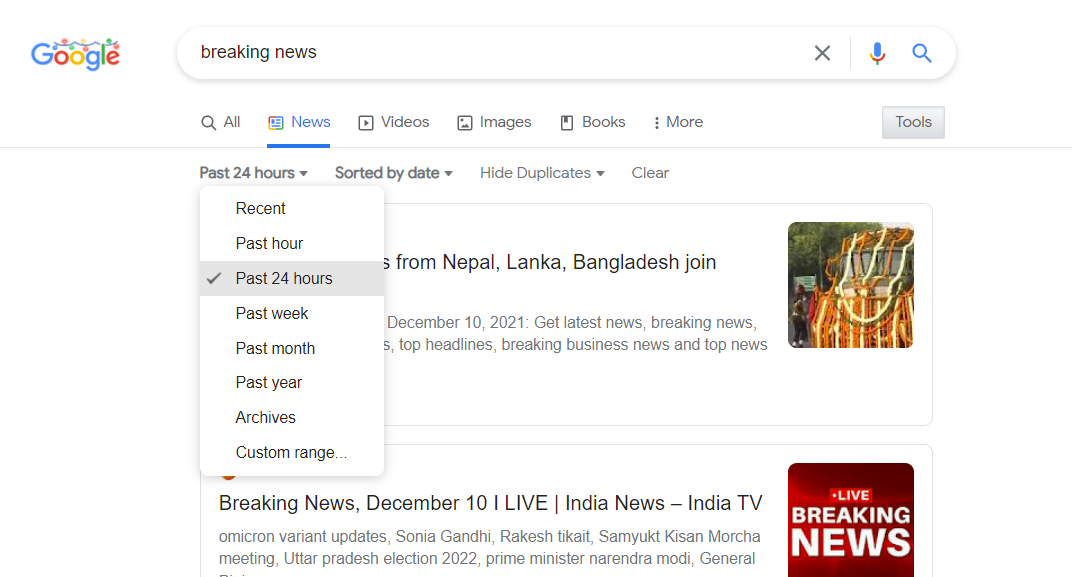This portrait-oriented photograph captures a screenshot of a Google search on a white background, with no clearly defined outer borders. At the top left corner, the Google icon is prominently displayed, modified to showcase the traditional blue, red, yellow, and green Google letters adorned with a string of multicolored lights, likely indicative of a festive, possibly Christmas-themed design. To its right is an elongated, oval-shaped search bar that contains the text "breaking news" in black font.

Beneath the search bar, there are various filter options, each accompanied by an icon. These include "All," "News," "Videos," "Images," "Books," and a "More" option, followed by a gray "Tools" button. A thin gray line demarcates this section, acting as a separator before displaying further filtering options. The first drop-down menu allows filtering by time, with the current selection being "Past 24 hours." It can adjust to other time frames ranging from recent to the past year. Next to it, another drop-down menu shows sorting options, with the current choice being "Sorted by date," followed by options to hide duplicates and a clear button.

Partially hidden by these drop-down menus is a link to a news story, starting with text concerning Nepal and Bangladesh, along with additional content that is obscured and a thumbnail image of an orange-hued vehicle. Directly below, another news article headline reads "Breaking News, December 10," followed by tags such as "live," "India news," and "India TV." This article also features a red image labeled "Live Breaking News."